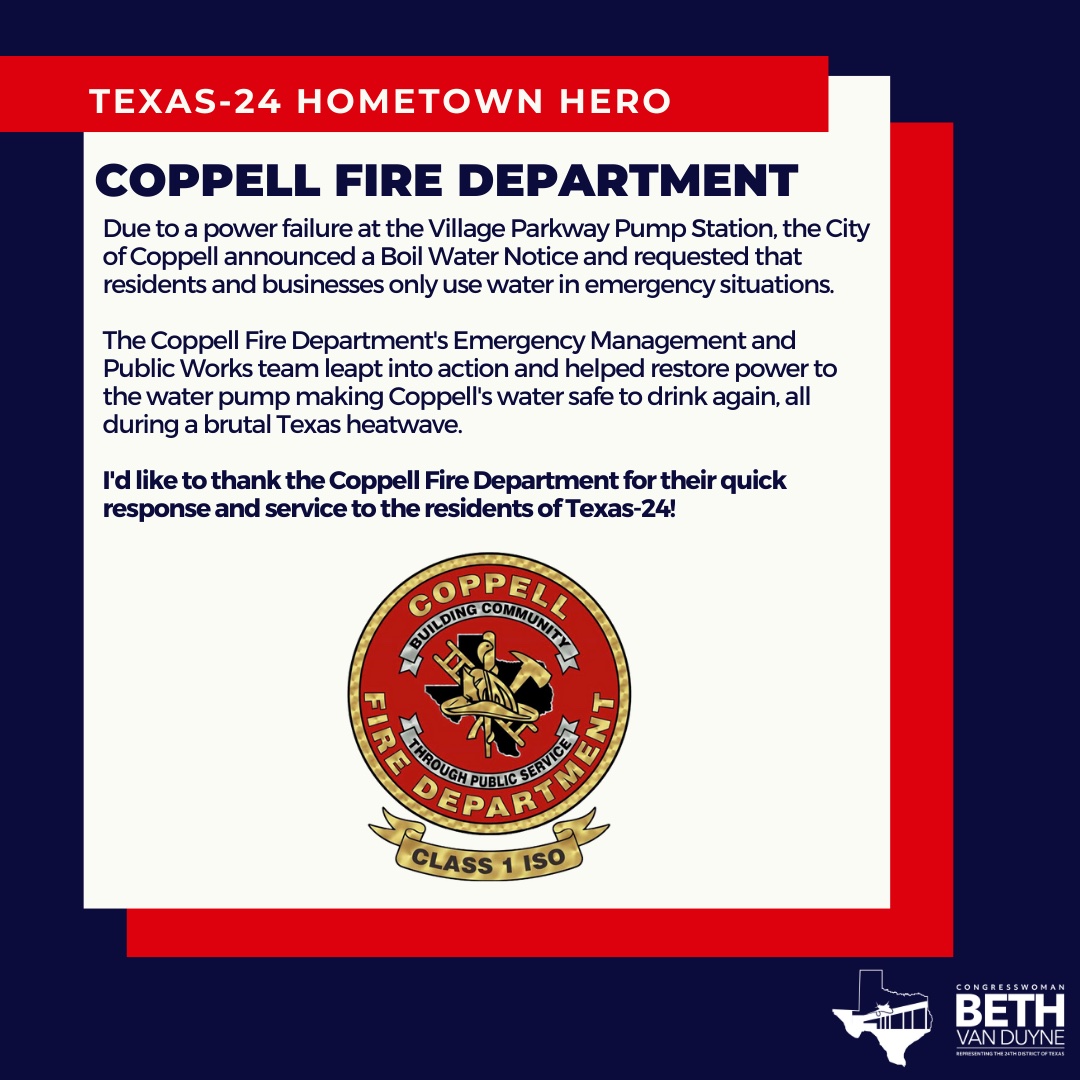The image is a digital poster, possibly designed for online sharing, issued by Congresswoman Beth Van Duyne of Texas. It announces the heroic actions of the Coppell Fire Department on a layered background, starting with dark blue, followed by red, and topped with white where the primary text is situated. At the top, a red bar features the title "Texas 24 Hometown Hero." The main white section highlights the Coppell Fire Department's swift response to a power failure at the Village Parkway pump station, which had led to a boil water notice during a severe Texas heatwave. The Fire Department, along with the Emergency Management and Public Works team, restored power to ensure the water supply was safe to drink, earning gratitude from the community. The poster concludes with a circular logo at the bottom showing "Coppell" at the top, "Fire Department" at the bottom, and a detailed depiction of Texas with fire insignia in the center, and a banner below that reads "Class 1150."